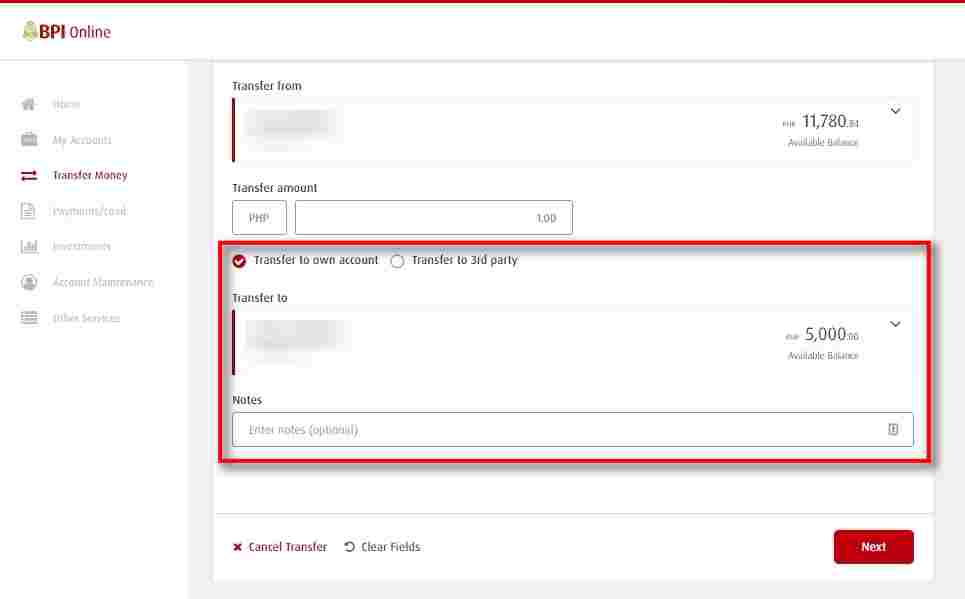The image depicts a bank's online transfer interface against a white background. At the top, there's a reddish line. Below it is a bell icon on the right side, colored yellow. The upper section also features the bold, reddish-brown text "BPI."

A thin gray bar separates this section from the next. On the left, there's a vertical gray bar listing menu options: "Home," "My Accounts," and in black text, "Transfer Money." Following this, in gray text, are the sections "Account Management," "Services," and several unreadable items.

The main section of the image features a white box bordered by two horizontal gray bars on the left and right sides. In black text within this box, it reads "Transfer From." Inside this area, some text is blurred out in gray. On the right side, it states "11,780" (presumably in PHP) as the "Available Balance."

Below, the section labeled "Transfer To" includes an area grayed out with the amount "5,000" specified. There's a drop-down menu showing "PHP" and another box displaying "$1." 

A reddish-brown checkmark indicates "Transfer to Own Account," while "Transfer to Third Party" is not checked. Additionally, there's a text box labeled "Notes," which is empty.

At the interface's bottom left, options "Cancel Transfer" and "Clear Fields" are available. The bottom right features a grayish-brown circle with the word "Next" in white text inside.